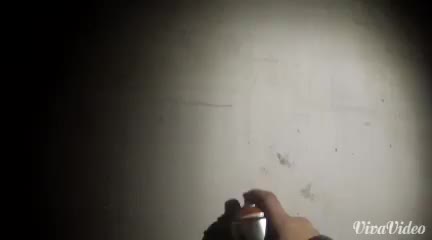In the image, we observe a hand holding a silver spray paint can with a white spraying part and an orange neck. The light brown hand is positioned at the bottom of the photograph, with the index finger placed on top of the spraying cap. The scene appears to be set in a dark environment, potentially night-time, illuminated by a flashlight that highlights a section of a grey, concrete wall. This spotlight effect reveals scuff marks and some black spots on the wall, contributing to the wall's worn appearance. Off to the left, the wall fades into darkness, while the right side remains more brightly lit. Notably, in the bottom right corner of the image, "Viva Vido" is written in white cursive text. Additionally, the can casts a shadow on the wall, reinforcing the setting's dramatic lighting.